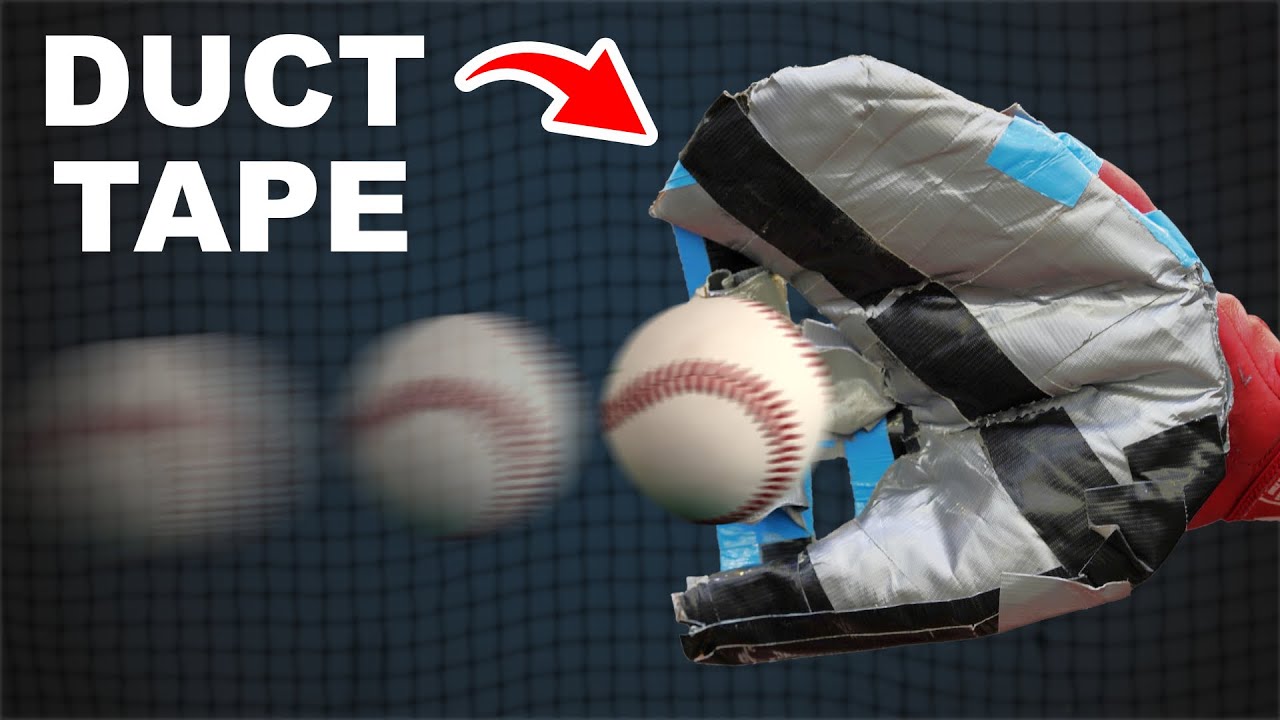The image features a creatively constructed baseball glove made entirely out of gray duct tape, prominently positioned on the right side. This unique duct tape glove is embellished with distinctive detailing: two black duct tape strips run from the fingers to the palm and from the thumb to the palm, while red duct tape accents the wrist. Blue webbing stretches between the thumb and fingers, enhancing its handmade aesthetics. The background is a dark gray, possibly representing a batting cage with netting, which appears to be made from blue painter's tape. A baseball, showcased with a dynamic motion effect, travels from the left towards the glove, its shadow adding depth to its swift movement. Just above, at the top left corner, bold white uppercase text reads "DUCT TAPE," complemented by a red arrow pointing directly at the glove. The overall composition, resembling a blend of photography and illustration, serves as an advertisement for duct tape, highlighting its versatility and creativity.